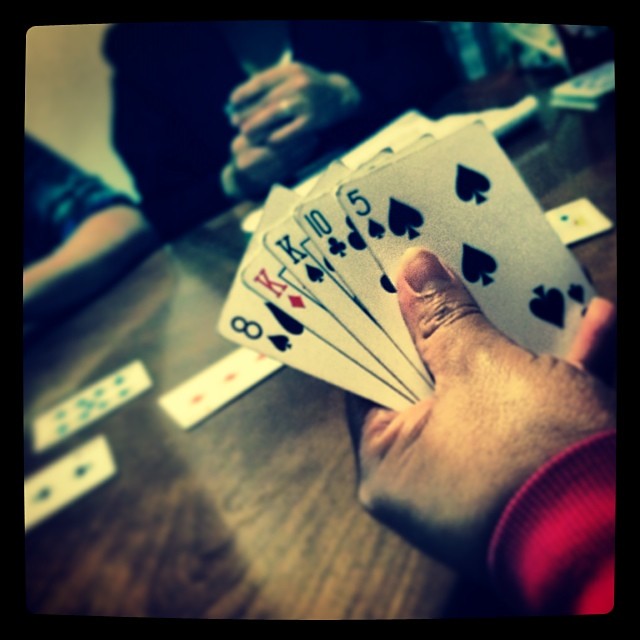A detailed point of view shot of a person playing cards shows their left hand entering from the lower right-hand corner, holding a hand of cards: the eight of spades, the king of diamonds, another king of diamonds, the ten of clubs, and the five of spades. In the foreground, these cards are held over a dark wooden table with a noticeable woodgrain pattern. The table also has several face-up cards, slightly blurred, but identifiable as the ace of spades, the ten of a black suit (possibly spades or clubs), and the three of diamonds. In the background, there are at least two other players. One is clearly visible, holding their hand of cards with both hands. This person is dressed in a black coat with a white shirt underneath. Adjacent to them, you can see the elbow of another individual, who appears to be wearing a blue flannel shirt rolled up to reveal their bare forearm.